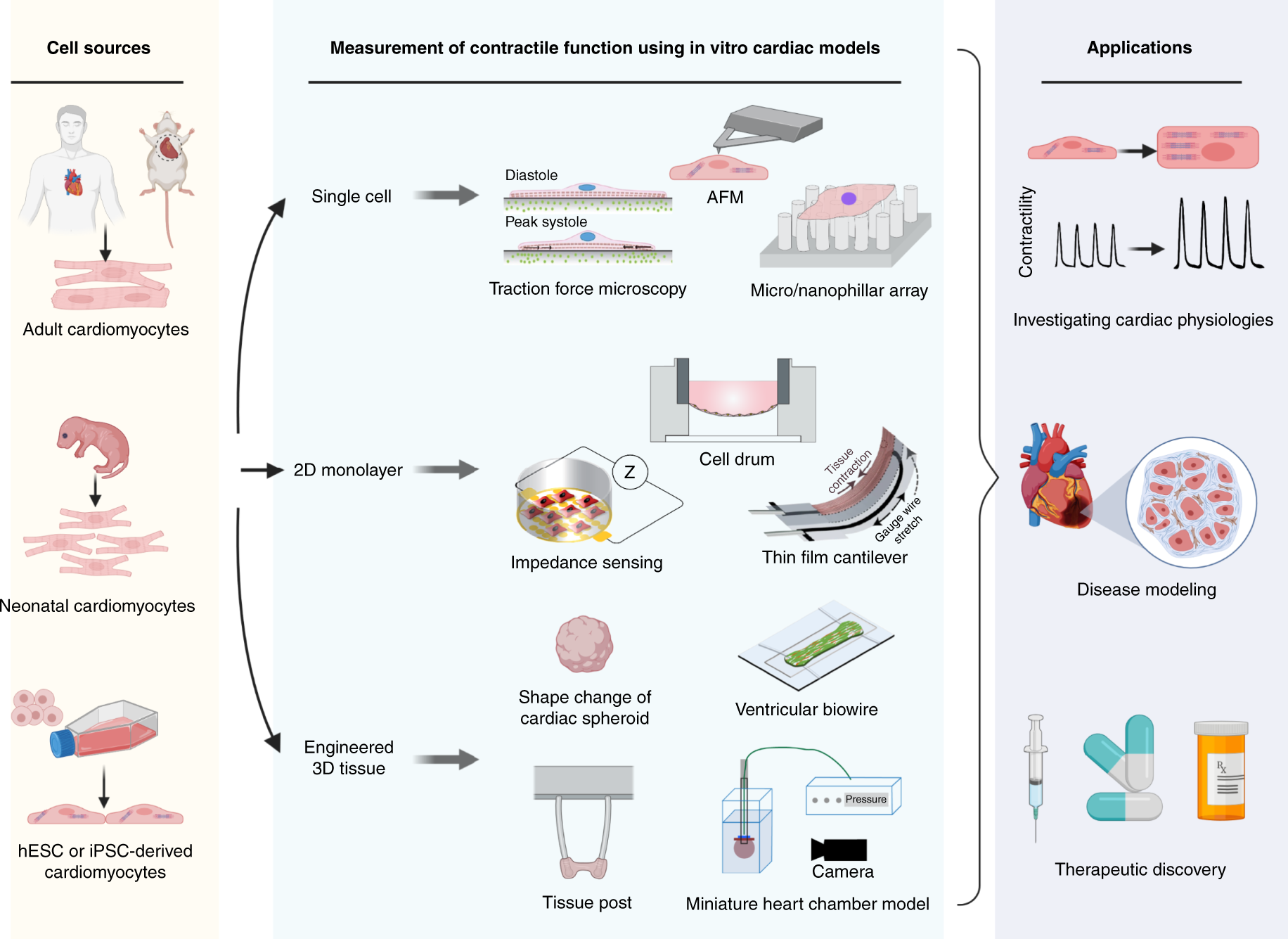The image is a detailed scientific diagram outlining the process of measuring contractile function in in vitro cardiac models. It is divided into three main sections: cell sources on the left, measurement methodologies in the center, and applications on the right.

The left panel, labeled "Cell Sources," features three types of cardiomyocytes: adult cardiomyocytes (depicted with an illustration of a man and a mouse showing their hearts), neonatal cardiomyocytes (represented with an embryo image), and HESC or IPSC derived cardiomyocytes (illustrated with a bottle containing pink liquid). Each cell type is accompanied by visuals showing their cellular structures.

The central section, titled "Measurement of Contractile Function Using In Vitro Cardiac Models," is further divided into three subsections:
1. **Single Cell:** This includes measurement techniques like diastole and peak systole visualized via traction force microscopy, AFM, and a micro-nanofiller array.
2. **2D Monolayer:** Methods here involve impedance sensing, cell germ, thin film cantilever with tissue contraction, and gauge wire stretch.
3. **Engineered 3D Tissue:** This employs tools like tissue post, tissue contraction, miniature heart chamber model, and ventricular biowire.

The right panel, labeled "Applications," lists three primary uses for these models: investigating cardiac physiologies, disease modeling, and therapeutic discovery. Each application aims to advance our understanding and treatment of cardiac conditions.

Overall, the diagram provides a comprehensive view of cell sources, measurement techniques for contractile function, and their practical applications in cardiac research.